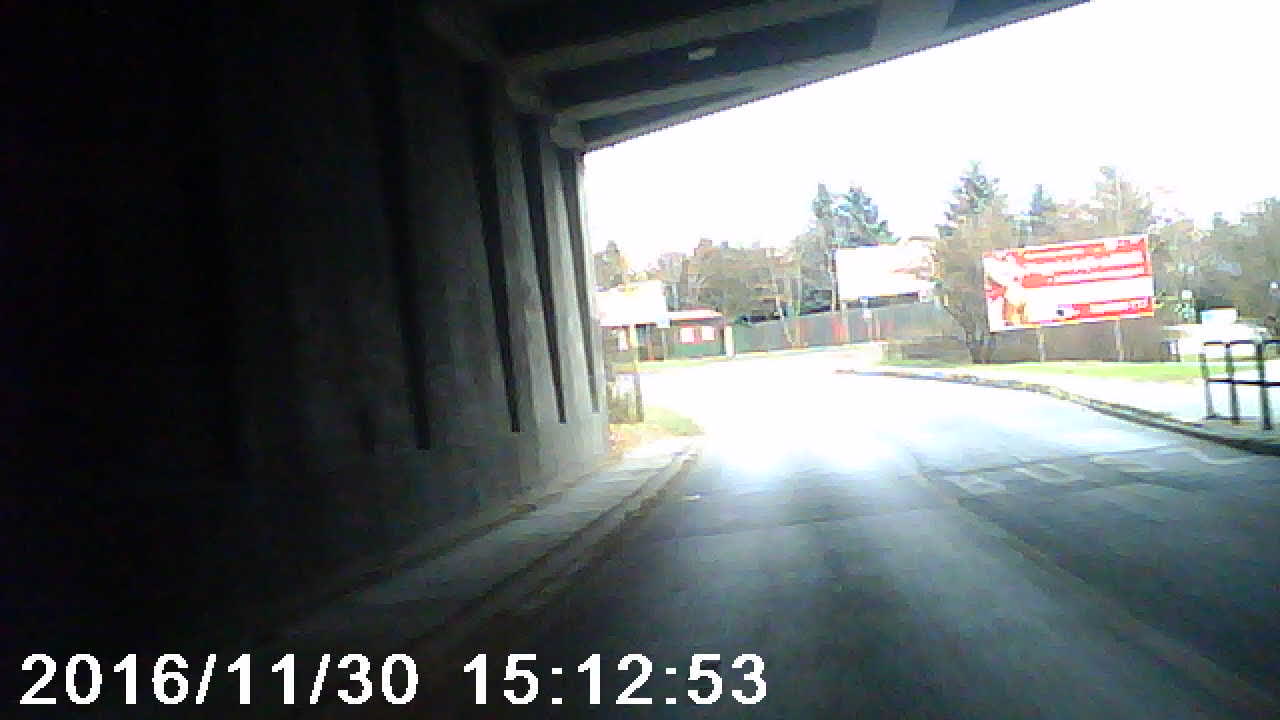A blurred photograph captures a roadway extending under a bridge. The bridge itself, with its gray stone wall prominently displayed on the left side, arches gracefully over the dark gray road. Above the road, the underside of the bridge can be discerned, though details are obscured by the blur. To the right, a black railing runs parallel to the roadway, accompanying light gray sidewalk pathways on either side. Past the bridge, the scene is washed in a bright white light, making it difficult to distinguish the buildings and fences that are vaguely visible in the background. In the distance on the right, a red rectangular billboard with indistinct white text adds a splash of color to the scene. Further back, a line of tall green trees, including bushy deciduous and evergreen pines, forms a vivid green backdrop. The sky above is an almost blinding white, contributing to the overall brightness and washed-out appearance of the photograph.